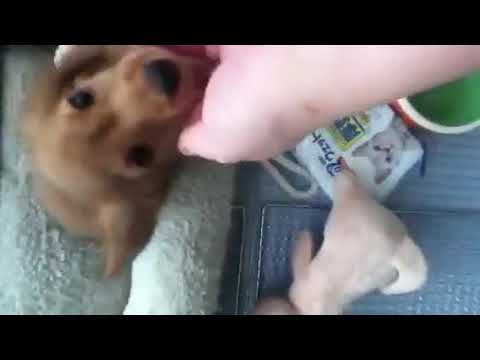In this photograph, a small rust-colored puppy with floppy ears, large black eyes, and a big black nose is lying in a gray dog bed on the left side of the image. The puppy appears to be looking up toward the camera, and a white hand is gently touching its face, possibly comforting it. One of the puppy's eyes seems injured. Surrounding the dog bed on the floor are a stuffed toy, a green cup with a white rim, and a package featuring a picture of a cat. The image is somewhat blurry, and two horizontal black strips frame the top and bottom of the photo.